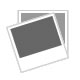The image depicts a shop window with a lit vintage advertisement for Double Cola. The window features sheer white curtains and a visible lit table lamp with a cream-colored shade on the left side. A maroon curtain, tied back, runs along the right side. The advertisement is a circular sign with concentric rings: an outer black ring, a white ring, a thin inner black ring, and a central red circle. In large, white bubble letters, it reads "Double Cola" around the red circle. Inside this circle, a white circle outlined in red contains an image of a red Coke bottle with "Double Cola" written in white letters. Above the bottle, in red text, it states, "Since 1933." A black wire suggests the sign can be illuminated at night. The intricate details and classic aesthetic evoke a nostalgic feel, highlighting the heritage of the Double Cola brand.